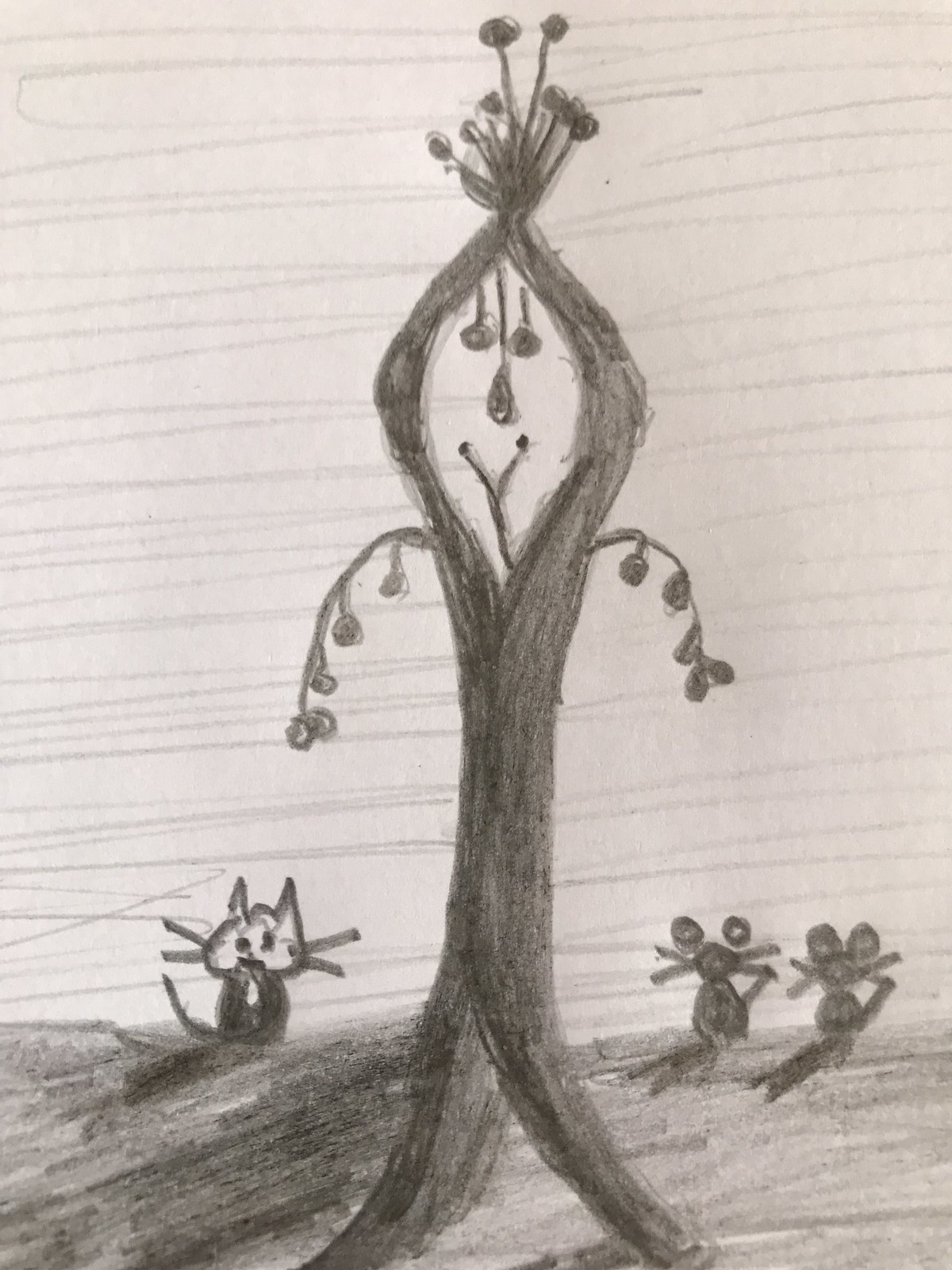This black and white drawing, rendered on white paper, features a striking central figure that extends from the bottom to the top of the image. The figure possesses elongated legs positioned to the left and right and stick-like arms adorned with round objects hanging from them. Its face is detailed with two eyes, a V-shaped mouth, and a nose, crowned with mind-like hair accented by bulbs at the top. To the left of the main figure, there's a small creature sitting on the ground, distinguished by its pointy ears.